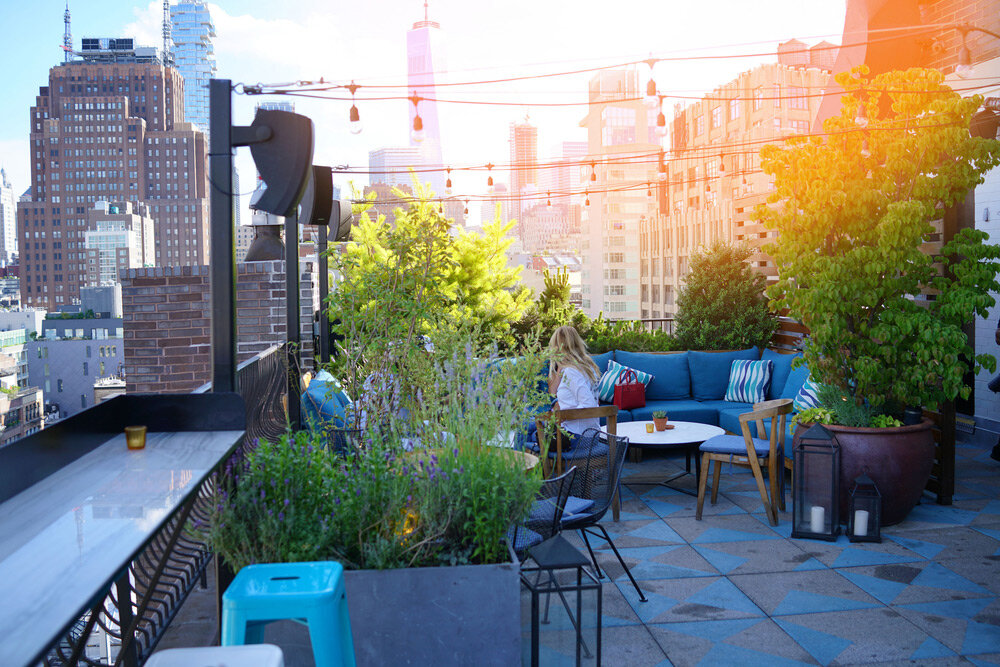This photograph captures a rooftop terrace perched atop a tall building, offering a stunning urban panorama filled with skyscrapers. The foreground hosts a meticulously designed open-air space adorned with a blue wraparound sectional sofa decorated with striped pillows in blue, white, and brown hues. A blonde woman with long hair, clad in a white shirt, sits in a wooden chair featuring a plush blue cushion that complements the sectional.

This outdoor oasis is enriched with various planters, including large rectangular ones and smaller pots, housing diverse plants and small trees that provide a refreshing burst of greenery. One prominent tree in a chocolate-brown planter stands tall, while other planters in gray concrete and clay dot the area, framing the space beautifully.

The deck's floor is an intricate assembly of gray tiles interspersed with blue triangular patterns, contributing an artistic touch. A sleek white table near the sectional holds a small glass and a cylindrical picture, with additional seating options like light brown wooden and black cushioned chairs arranged thoughtfully around it. There are small candles in glass holders scattered around, contributing to the cozy ambiance.

Above, string lights crisscross the sky, casting a warm glow as evening approaches, complementing the breathtaking sunset that bathes the cityscape in hues of orange and red, while part of the sky remains a serene blue. Additional elements like a bar with stools facing the edge of the balcony, small speakers on posts supporting the string lights, and a patterned blue and gray tile floor enhance the space’s charm. Overall, this rooftop patio is both a tranquil refuge and a nod to the dynamic city surrounding it.